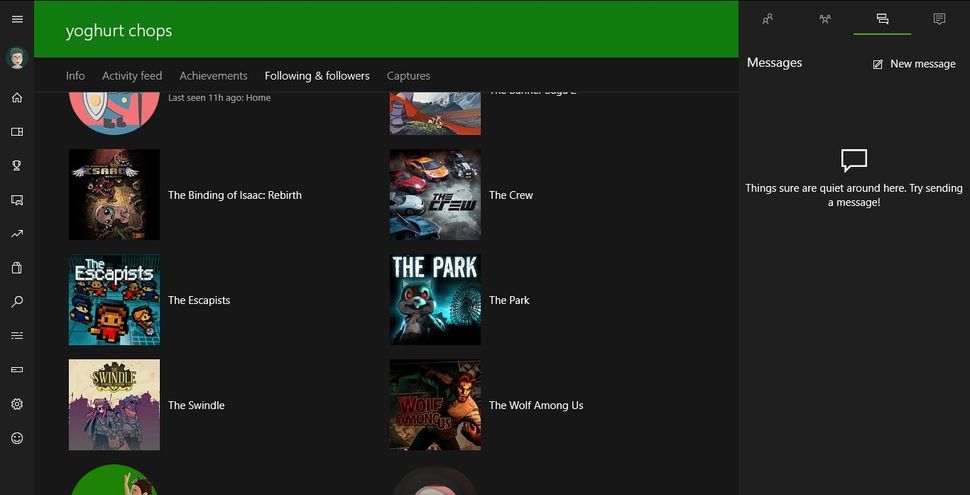The image showcases a detailed view of a gaming website's user interface. At the top of the screen, there is a dark green bar featuring the website's name in white letters, "Yog Heart Chops". Directly below, a black navigation bar provides options such as Info, Activity Feed, Advertisements, Achievements, Follow, Following, Followers, and Captures.

On the left side, there is a vertical sidebar with various icons for navigating different sections of the website, including Home, Search, and more.

The central portion of the screen is dominated by a display of game titles with their cover images. The layout presents five games in two columns:

- The left column contains:
  1. A game title that is unreadable
  2. Another unreadable game title
  3. The Binding of Isaac: Rebirth
  4. The Escapists
  5. The Swindle

- The right column contains:
  1. A game title that is unreadable
  2. The Crew
  3. The Park
  4. The Wolf Among Us
  5. A game title that is unreadable

The bottom part of the screen features a message section with the prompt "Sure are quiet around here. Try sending a message", inviting users to engage by sending new messages.

Finally, at the very top right of the interface, there are clickable icons for additional navigation options within the website.